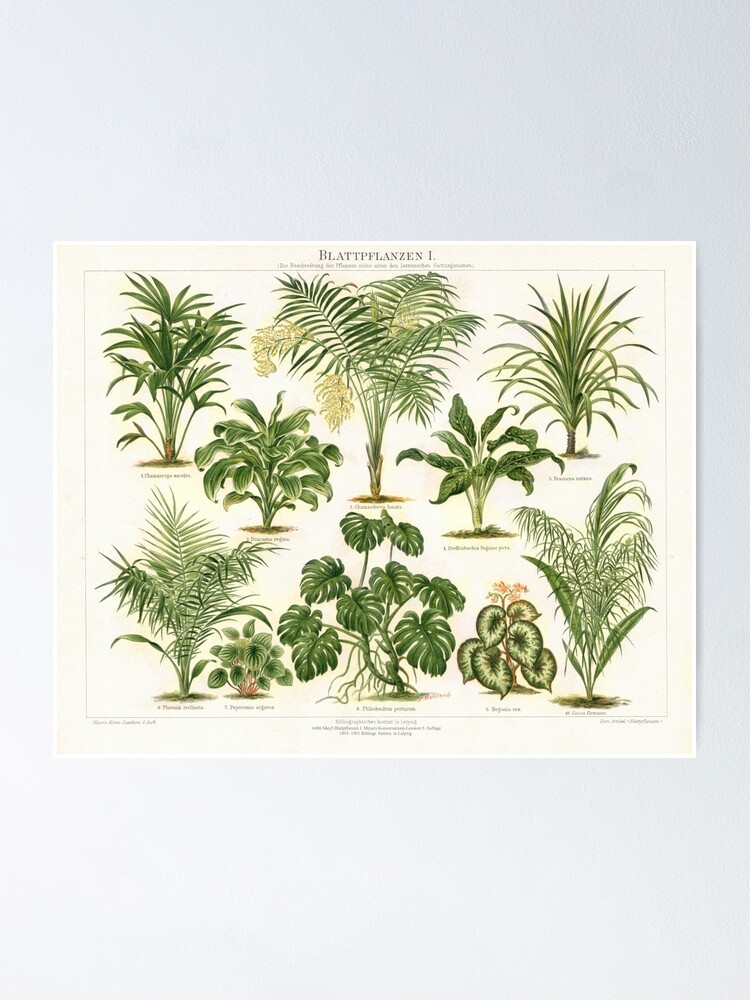This image is a detailed botanical art illustration in landscape orientation, depicting various indoor plants. The background is a cream color, set against a grayish-blue wall. Across the top, "BlattPlanzen 1" is written in bold, black, all-caps text, with some illegible writing underneath. The illustration features ten different plants, each with names labeled in small, black text underneath that are unreadable. The plants are arranged in three rows: three across the top, two in the center, and five along the bottom. The plants on the left side have taller leaves, those in the middle include more flowering and palm-like varieties, and the right side displays spiny plants. Among the bottom row, the plants range from spiny and thick-leaved to stubby with circular leaves, and a variety with white and green leaves in the bottom right. The leaves are mostly dark green with occasional brown and yellow highlights, lending to the realism and detail typical of botanical illustration. The illustration captures the greens, tans, and whites of the different plant species beautifully.